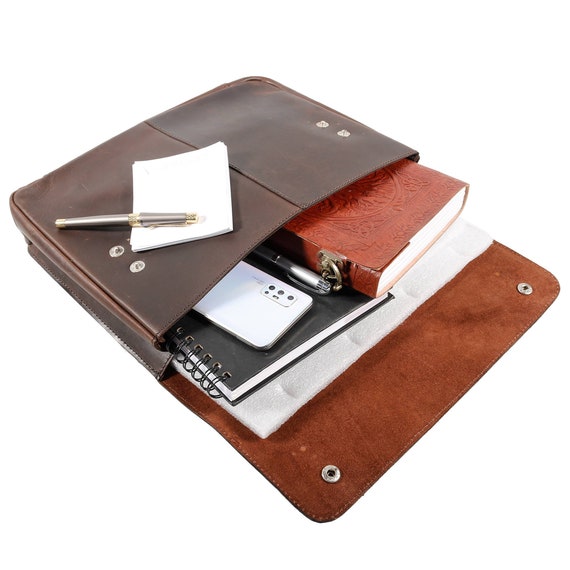This photograph features an open brown leather satchel, elegantly laid against a stark white background. The satchel, positioned with its open flap facing the bottom right corner, reveals a rich, felt-lined interior secured by silver metal snaps. Inside the satchel, there is a brown hardcover book, a black spiral-bound notebook, and a white smartphone, its camera visible. A silver and gray pen rests on top of the notebook, while a larger white mailing envelope is partially tucked beneath the assorted items. Spread across the outside of the satchel's flap is a small folded piece of paper, accompanied by a silver pen with golden tips, completing the meticulously arranged contents of this sophisticated carrying case.